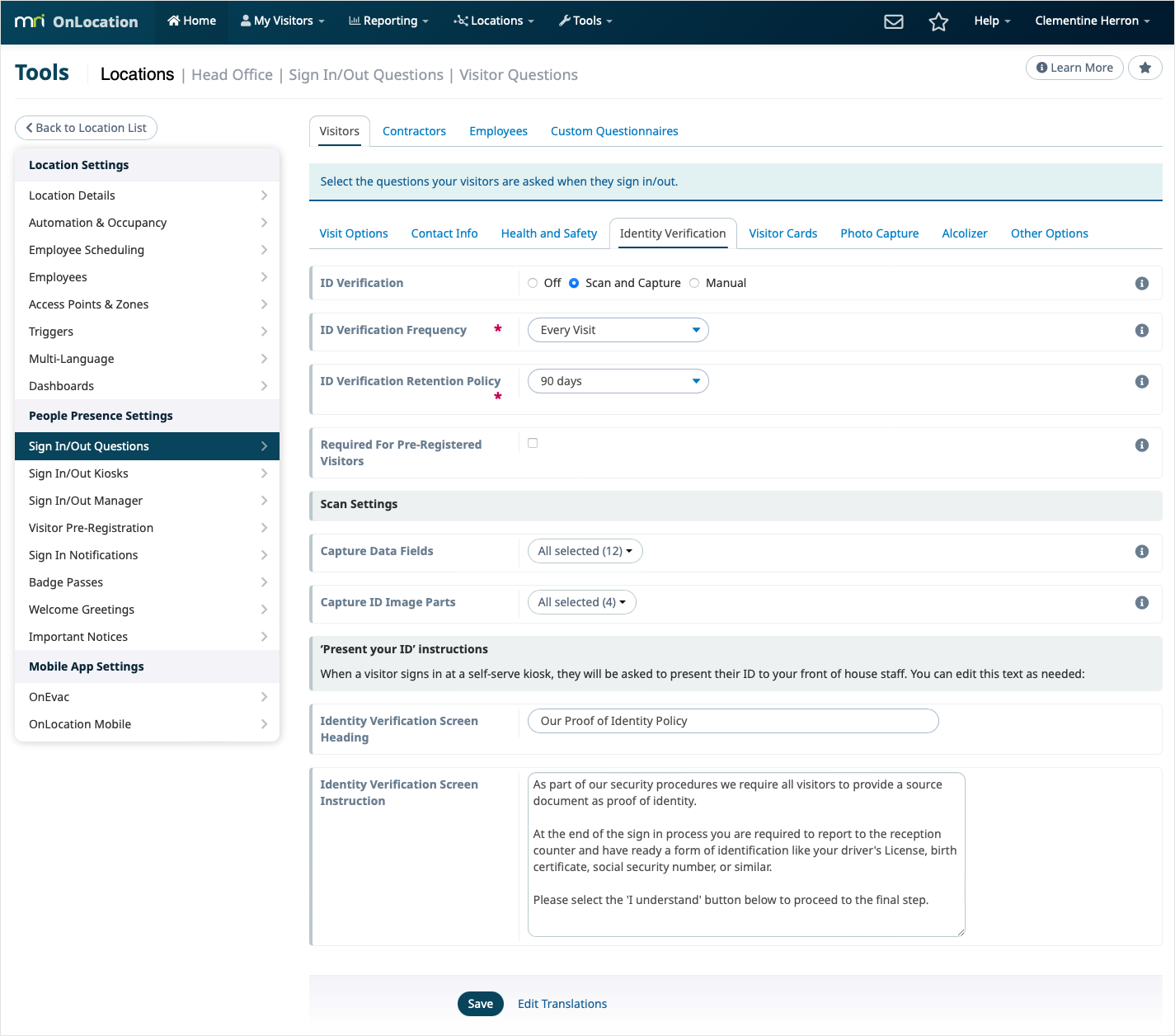The image depicts the user interface of an MRI monitoring site, featuring a recognizable logo with the letters "MRI" in lowercase on the header bar. The header includes various menu buttons such as "Home," "My Visitors," "Reporting," "Location," and "Tools." On the far right, icons for email, favorites (star icon), and a help menu tab are visible, alongside the user profile named Clementine Heron.

Below the header, there's a submenu including buttons for "Tools" and a "Location" menu showing options like "Head Office," "Sign-In/Out Questions," and "Visitor Questions." To the right, there’s a "Learn More" button and a gray star icon, representing an additional interactive element.

On the left, a detailed column lists several categories including "Location Settings," "Location Details," "Automation," and "Occupancy." Further down, settings for "People Presence" and a highlighted section for "Sign-In/Out Questions" are displayed. A bar menu appears below this, providing options for "Sign-In," "Sign-Out," "Kiosk," and other functionalities.

To the right of this, menus for "Site Visitors," "Contractors," "Employees," and "Custom Questionnaires" are clearly laid out, ensuring comprehensive access to various user and visitor management tools. The interface is designed to facilitate easy navigation and detailed monitoring of site operations.